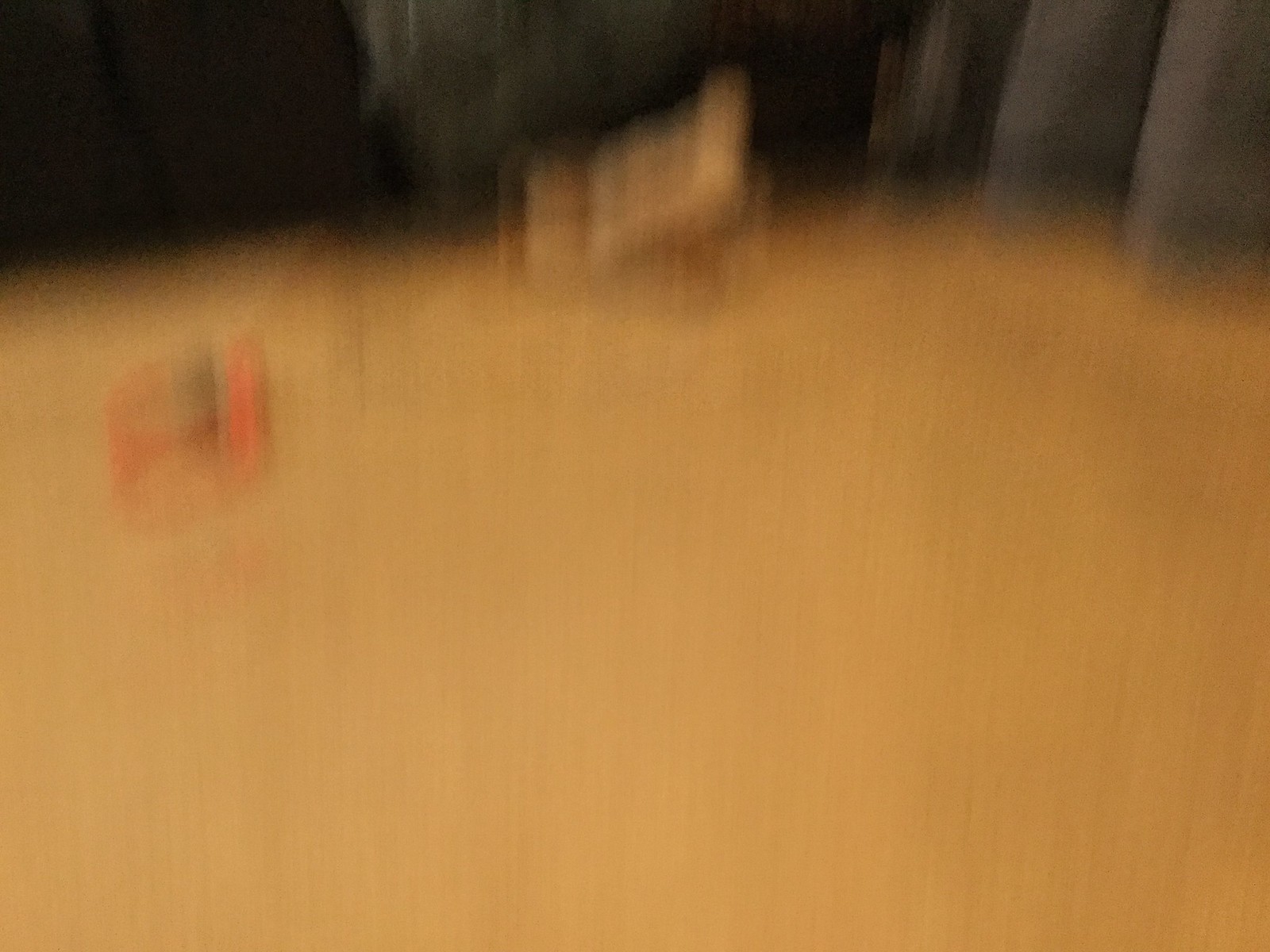The image is extremely blurry, predominantly shaded in beige or tan hues. It depicts what might be a living room scene, with a large area covered by dark beige or tan carpet. On the right side, there appears to be a gray piece of furniture, possibly a couch, suggested by its vertical lines akin to the back of a couch. In the middle, there is a gray, indiscernible object that might be an animal. A gray wall is perceived in this area, extending about a third of the way across the image, with what seems to be a small, hump-like structure or ramp higher on the right side. Just inside from the left, there's a hint of a crack in the wall.

To the left side of the image, potentially another piece of furniture in a brownish shade is visible. An open book possibly sits atop this, which one might assume rests on a coffee table although the table itself is not distinctly visible. Near this book is a small red blob, its identity unclear. Directly behind these items in the background, there are some dark areas in various shades of grays and browns, creating an indistinct mix of dark whites and gray.

Additional details include two small, gray pillars on the darker side of the photo, and just below the left edge is a small square marked with orange and black. The image, while strikingly vague, presents a highly abstracted and indistinct interior scene framed by pastel and darker neutral tones.